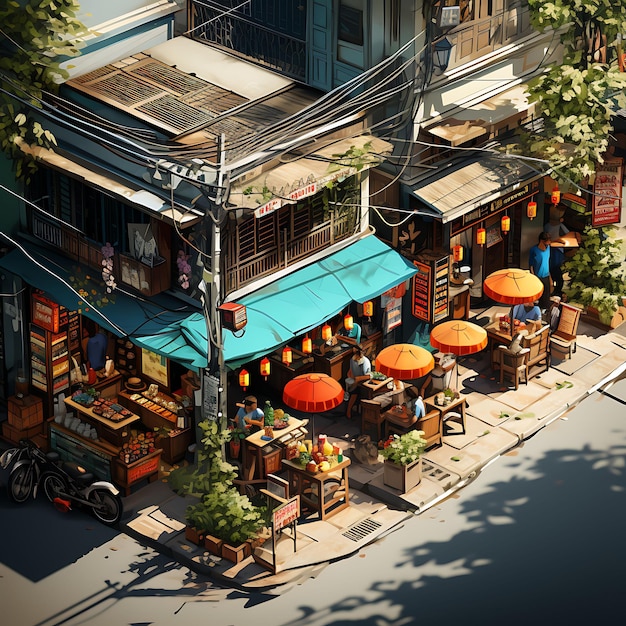The image depicts an artistic rendering of a vibrant street corner in a South or East Asian market, likely indicative of a Vietnamese, Indonesian, Thai, or possibly other Asian locales. The scene is dominated by four bright orange umbrellas shading small tables on the sidewalk, each surrounded by people enjoying their meals. Multicolored food items are visible, adding a burst of color and life to the scene. To the left, near the bottom of the image, parked motorcycles line the street, next to a fixed, outdoor food stand with a blue canopy above it.

The decorative elements include a series of yellow lanterns with red tops and dangling cords hanging from a teal-turquoise overhang, enhancing the festive atmosphere. This overhang belongs to a permanent structure that resembles a hybrid between a street food cart and a small restaurant, which is adjacent to a more industrial-looking building with loose power lines extending above, typical of the region.

A large tree casts a shadow on the street, hinting at a sunny day with the sunlight illuminating various elements like the tops of buildings and umbrellas. The image combines a photo-realistic quality with elements of watercolor and smudge effects, giving it the appearance of a detailed painting or an AI-generated piece of art. The perspective is from an upper-level building looking down, capturing the entire bustling corner, complete with square tables, green-leafed planters, and even a drain on the sidewalk corner.